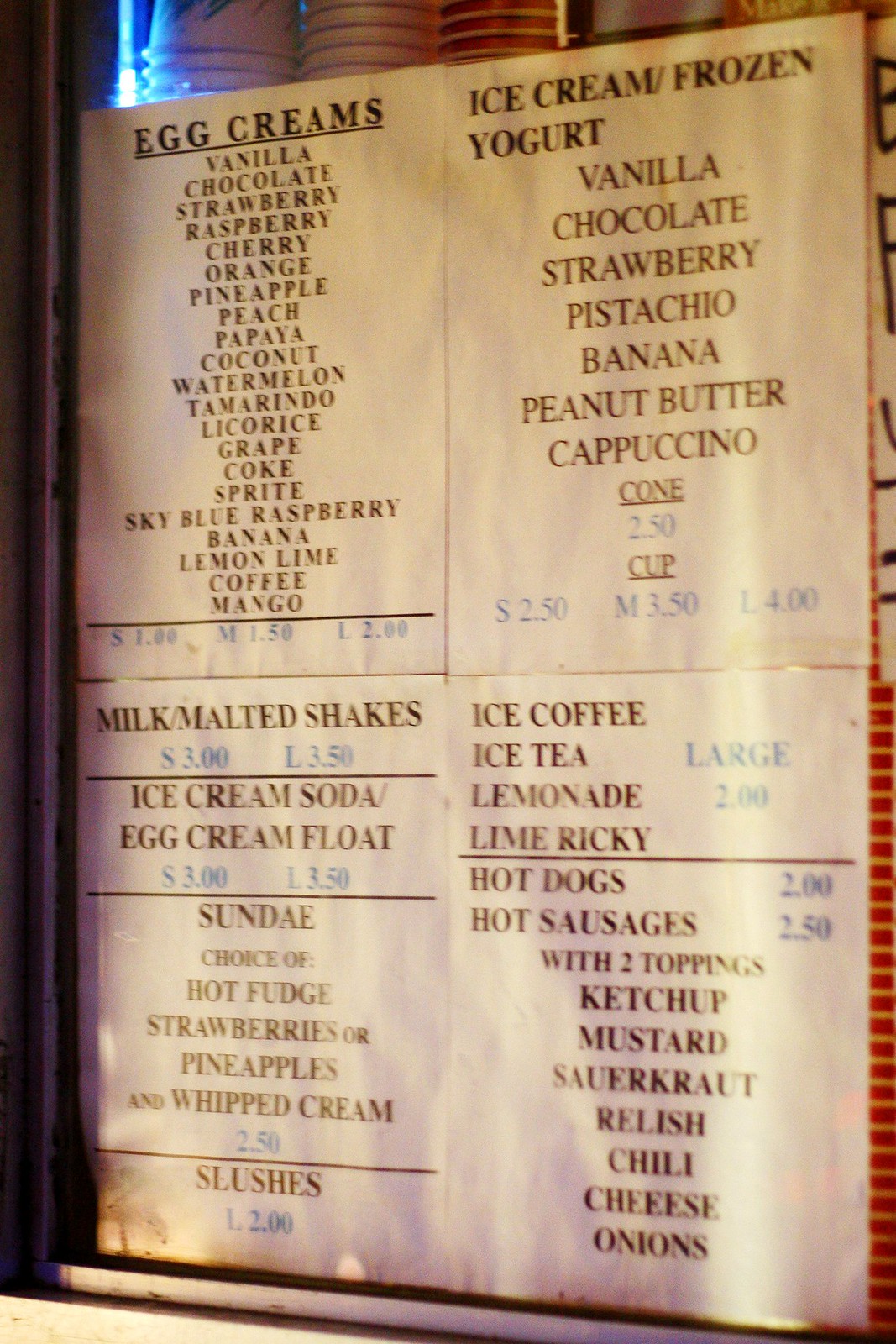The image depicts a detailed menu from a dessert or coffee shop, affixed to a glass window using four different pieces of paper arranged in groups of two, one above the other. Here's an enhanced and organized description of the menu items:

### Top Left Menu:
- **Egg Creams** (underlined)
  - Flavors: Vanilla, Chocolate, Strawberry, Raspberry, Cherry, Orange, Pineapple, Peach, Papaya, Coconut, Watermelon, Tamarind, Licorice, Grape, Coke, Sprite, Sky Blue, Raspberry, Banana, Lemon, Lime, Coffee, Mango.
  - Prices: Numbers are blue and somewhat faded.

### Bottom Left Menu:
- **Milk/Malted Shakes**
  - Price: $3.00 (blue; left side) and $1.25 (blue; right side; somewhat faded)
- **Ice Cream Soda/Egg Cream Float**
  - Price: $3.00 (left) and $3.50 (right)
  - Black bold line separator
- **Sundae**
  - Choices: Hot Fudge, Strawberries, or Pineapples with Whipped Cream
  - Price: $2.50
  - Brownish black bold line separator
- **Slushies**
  - Price: $1.20

### Top Right Menu:
- **Ice Cream/Frozen Yogurt**
  - Flavors: Vanilla, Chocolate, Strawberry, Pistachio, Banana, Peanut Butter, Cappuccino
  - **Cone** (underlined)
    - Price: $2.50
  - **Cup** (underlined)
    - Small: $2.50
    - Medium: $3.50
    - Large: $4.00

### Bottom Right Menu:
- **Iced Coffee/Iced Tea**
  - Large: $2.00
  - Flavors: Lemonade, Lime Ricky
  - Separator line
- **Food Items**
  - **Hot Dogs**
    - Price: $2.00
  - **Hot Sausages**
    - Price: $2.50
    - Includes two toppings: Ketchup, Mustard, Sauerkraut, Relish, Chili, Cheese, Onions

The detailed arrangement and faded elements suggest a nostalgic and possibly well-loved establishment, offering a variety of desserts and snacks to its patrons.